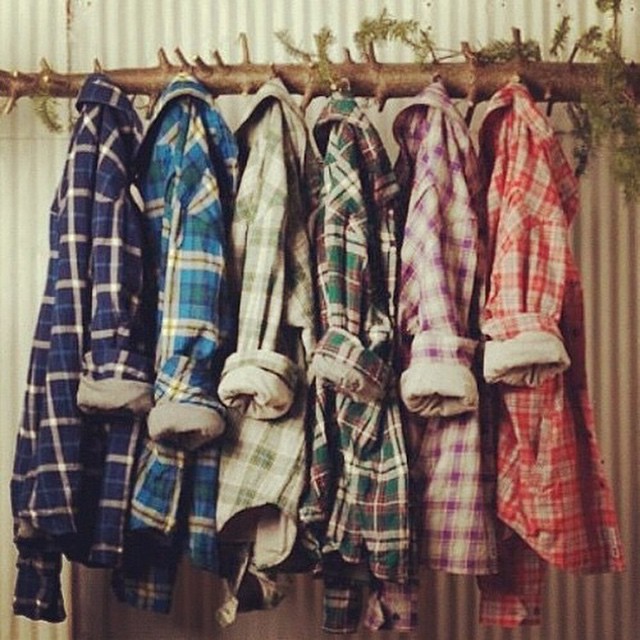This indoor photograph captures six colorful plaid robes hanging from a horizontally positioned, roughly cut pine tree branch, which runs across the upper part of the image. The branch, adorned with a few remaining needles and irregularly pruned stubs, acts as natural hooks for the robes. Each robe faces rightward, with sleeves cuffed to reveal their inner linings. The robes, part of a cohesive set despite their color variations, exhibit patterns of dark blue and white, light blue and green, very light green and ivory, dark green with red and ivory, ivory with bright purple, and red with white. They hang against a backdrop of vertically striped white and gray wallpaper, adding a touch of rustic charm to the otherwise industrial setting.